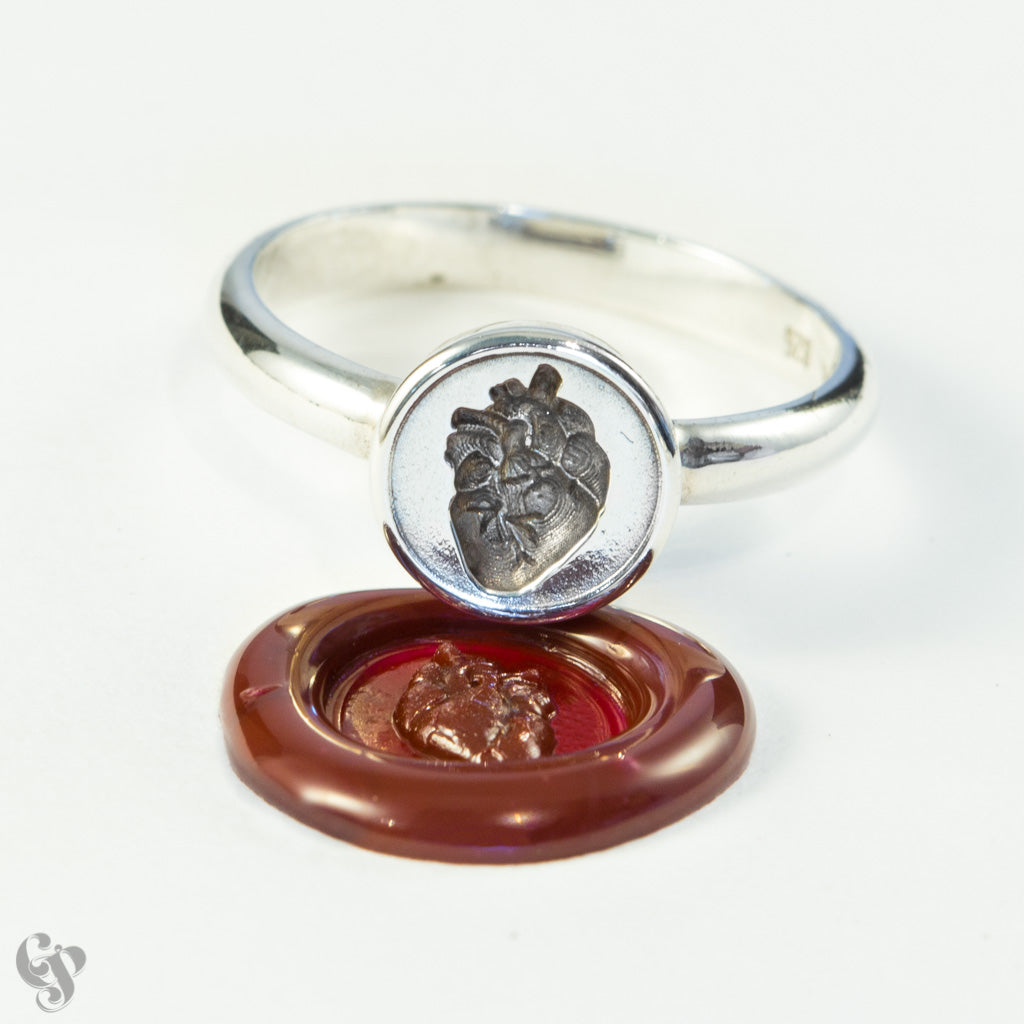The image depicts a close-up view of a silver ring placed centrally against an off-white background. The ring is a simple silver band with a circular face that features an intricate imprint of a human heart, rather than a gemstone. The environment suggests direct lighting, as evidenced by a shadow cast to the right. The ring is positioned upon a reddish-brownish wax seal, which clearly shows the same heart design imprinted by the ring's stamp. In the lower left corner of the image, there is a grey and white insignia, possibly saying "CP" in calligraphy, although the exact details of the logo are ambiguous. The ring shows a "925" mark, indicating its authenticity as real silver.